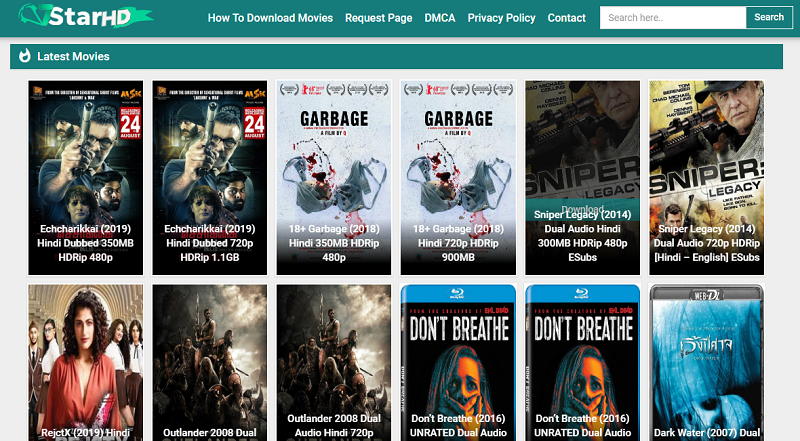The top of the image features a dark blue header displaying a logo. Below the header is a distinctive teal banner with a ribbon element, prominently labeled "Star HD." On the right side of the banner, there is a navigation menu with several clickable options: "How to Download Movies," "Request Page," "DMCA," "Privacy Policy," and "Contact."

Directly beneath the navigation menu is a search bar with a search button on its right side. A smaller dark blue rectangular area labeled "Latest Movies" is positioned below this. Under the "Latest Movies" banner, there are six movie thumbnails arranged in two rows. 

The two thumbnails on the top left display a title that's difficult to read, potentially obscured, and labeled inconsistently with "in shower okay." Next to these, on the right, are two thumbnails titled "Garbage 18+ (2018)." The last two thumbnails on the right are labeled "Sniper: Legacy (2014)."